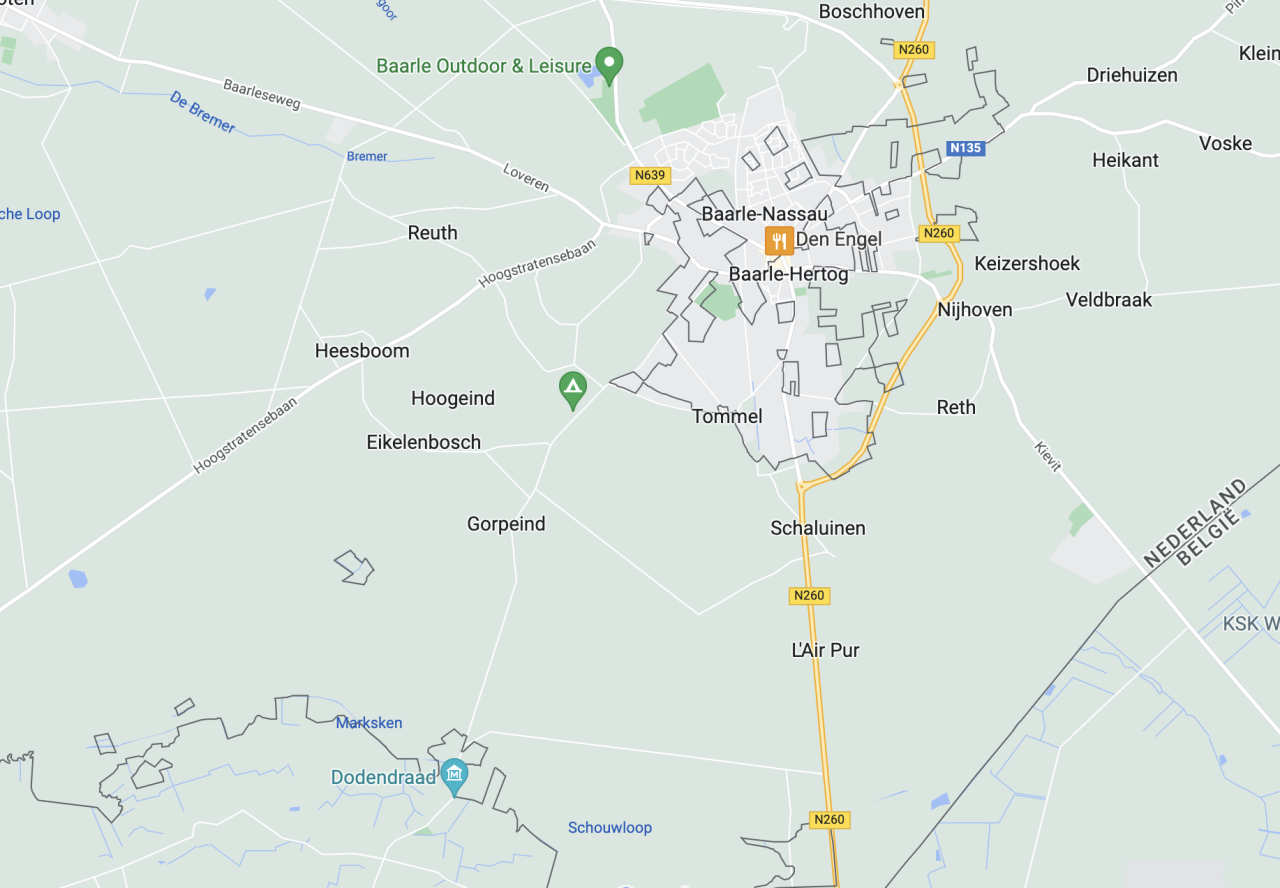This digital map screenshot appears to depict a small European region, possibly in the Netherlands, based on the labeling of towns and roads. The central town of focus is Barle-Nassau, with the name "Barley Hertog" also visible, suggesting a border area since Barle-Nassau is known for its complex border with Belgium. The map features a prominent yellow road labeled N260, which runs along the outskirts of Barle-Nassau and continues down the map's center axis. Roads and labels are displayed on a gray background with white lines for the roads. Among other marked locations, there is a selected site labeled "Barley Outdoor and Leisure" with a green marker, situated near a small lake. On the far right, a larger font labels "Nederlandmeestje," possibly indicating a major road or area. Additional towns like Tommel, Reth, Voske, and Lapeur are also marked, enhancing the map's detailed representation of the region.